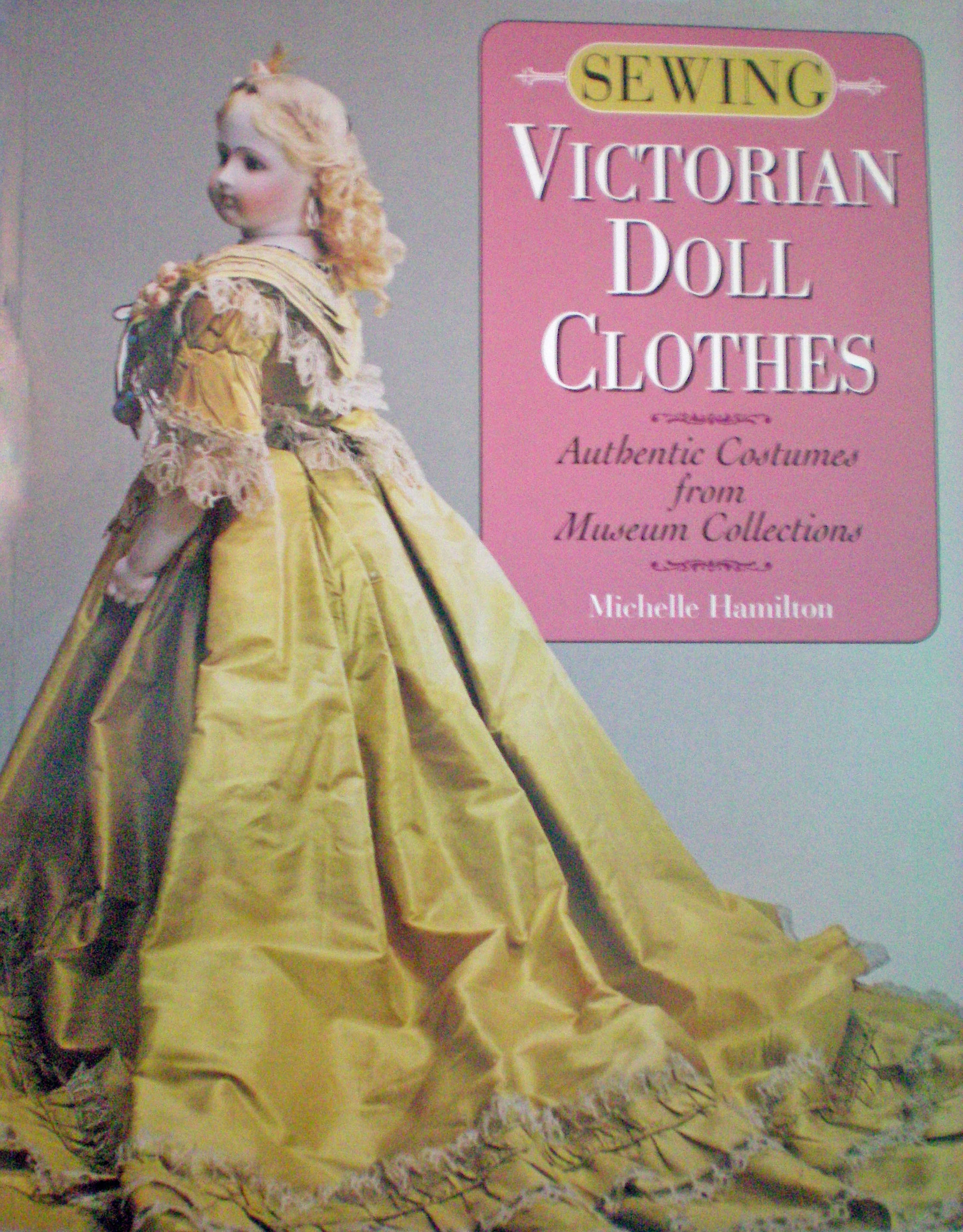This photograph depicts the cover of a book with a bluish-gray background. On the top left side of the cover, there appears to be some water damage that has caused the gray color to look slightly washed out. Central to the image is an ornate porcelain doll featuring reddish-blonde hair styled with a floral headpiece. The doll is dressed in a long, elaborate Victorian ball gown in a dull mustard yellow color, adorned with intricate lace and ruffles on the sleeves, back, and bottom hem. The doll also has rosy cheeks and holds a flower decoration on its chest.

To the upper right corner of the cover is a prominent pink rectangle. At the very top of this rectangle is a small yellow oval with the word "Sewing" inscribed in it. Beneath this in regular white font are the words "Victorian Doll Clothes," followed by "Authentic Costumes from Museum Collections" written in black. At the bottom of the pink rectangle is the author’s name "Michelle Hamilton" in white text.